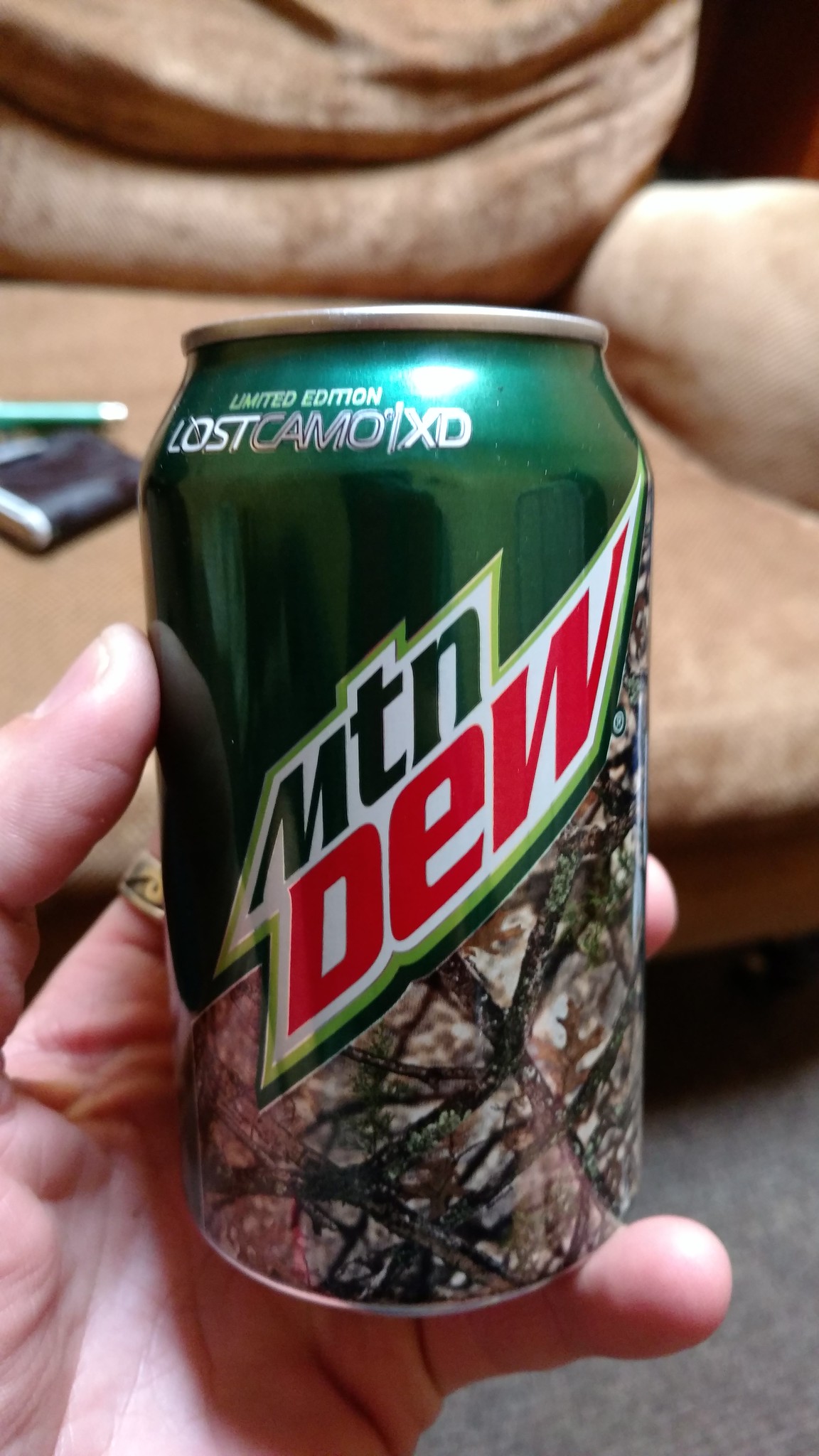A detailed photograph showcases a person holding a limited edition Mountain Dew can with their left hand. The can features a distinctive design, with the words "MTN Dew" emblazoned in a dark green and red font, set against a white background. Above the logo, the can reads "Limited Edition Lost Camo XD" in silver font. The lower half of the can is decorated with a camouflage pattern composed of various shades of brown, mimicking a forest floor with branches and leaves. The person's hand, specifically the thumb, pinky, and parts of the ring and pointer fingers, is visible. The pointer finger sports a gold ring adorned with circular designs. Behind the individual, a well-worn, plush tan armchair with visible wooden base peeks through, sitting atop dark gray carpet. Some additional items, including a green pen and possibly a wallet, rest on the seat of the chair.